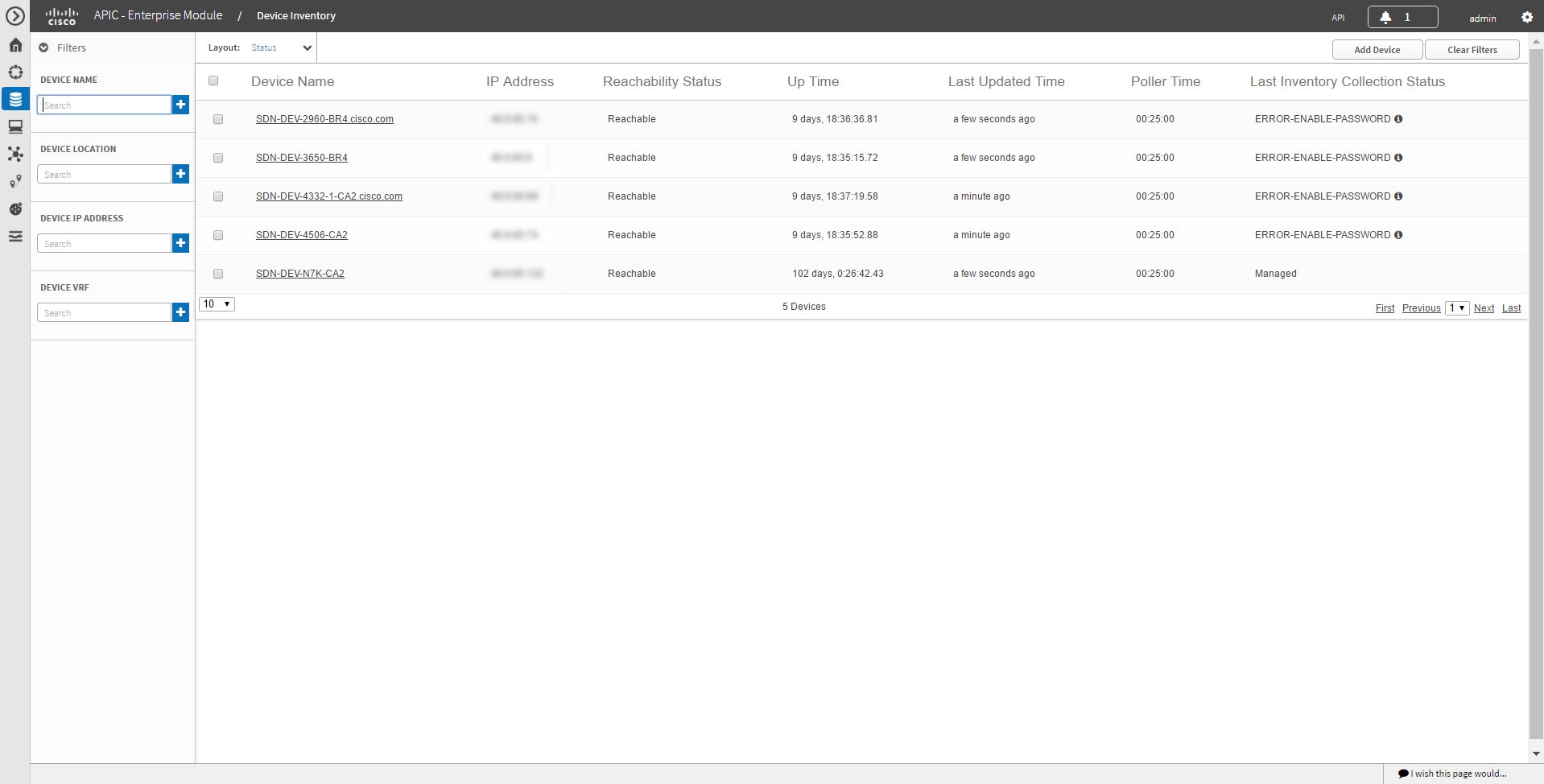This image displays a sophisticated directory interface, prominently featuring a black-bordered top banner. The header in this banner is partially obscured, but it clearly includes the key term "Device Directory." Notably, the Cisco logo is visible alongside the title "APIC L" followed by "Module/Device Inventory."

In the left sidebar, several icons are neatly arranged, the first of which is a home icon, followed by a star icon. The purpose of the remaining five icons is not discernible from the image. 

The central section of the interface is tabbed, with one tab currently active. The main content area beneath contains several filter boxes identified by clear labels paired with plus signs. Although the full text isn’t entirely legible, the first filter box appears to pertain to "Device Name," followed by "Device Location," "Device IP Address," and "Device VWP."

A table occupies much of the screen, listing five entries under "Device Name." Each device entry is accompanied by its corresponding "IP Address." Adjacent columns provide further details, such as "Reachability Status," "Uptime," "Last Updated Time," "Poller Time," and "Last Inventory Collection Status."

Above this table, there are two tabs whose labels are indiscernible. Returning to the black banner at the top, a notification icon is visible, indicating one unread notification.